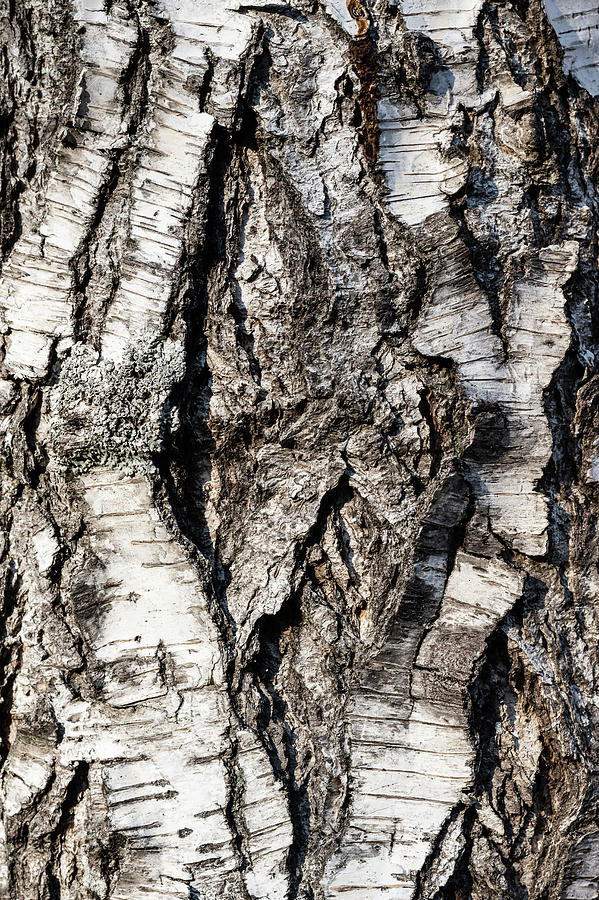This photo is a long, vertical, triangular close-up of tree bark, filling the entire frame. It shows a highly textured and layered surface with distinct vertical lines running from top to bottom. The bark features a mix of dark browns, grays, and a silvery white, likely sun-bleached in some sections, giving parts of the bark a light gray to white appearance. The central section of the bark appears more solid, while the sides have slash-type markings that emphasize the rough texture. There is no text or other objects present in the image; it's solely focused on the intricate details and natural patterns of the tree's bark, which gives a sense of an old, mature, and large tree.